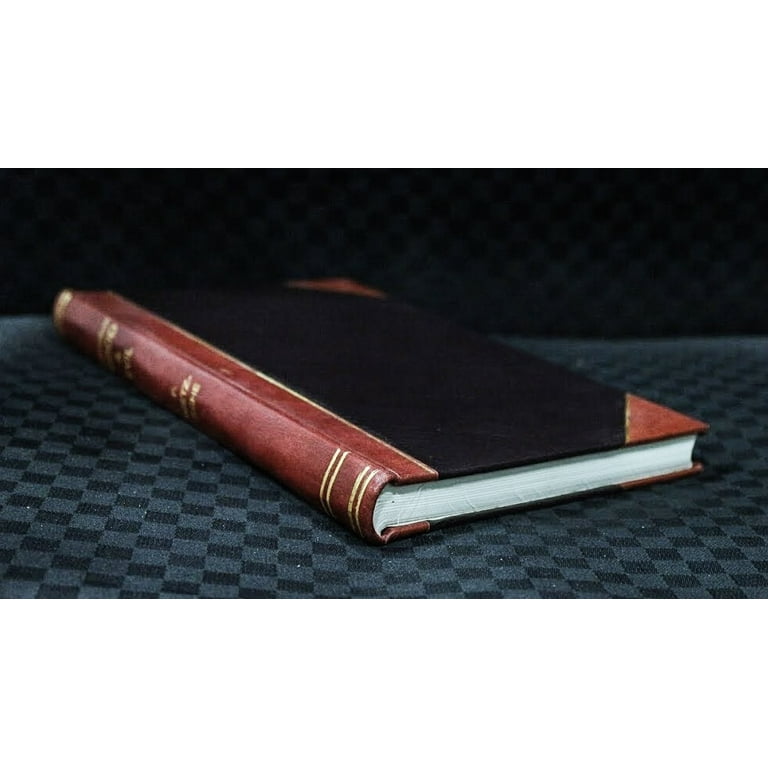This photograph captures a book with a vintage aesthetic, modeled against a dark blue checkered backdrop that may be a cloth or carpet. The primary focus remains on the book due to the pure black background surrounding it. The book’s cover is predominantly a plain black or very dark navy blue shade, featuring crimson red, triangular corners add to its intriguing design. The spine is adorned with gold lines and blurred golden text, likely indicating the title and author. Despite some blur, the gold embellishments suggest an air of elegance. The book is relatively thin and its pristine pages remain bright white, suggesting it has been well-preserved. There are no visible imperfections, and the absence of a title on the front cover enhances its mysterious allure.